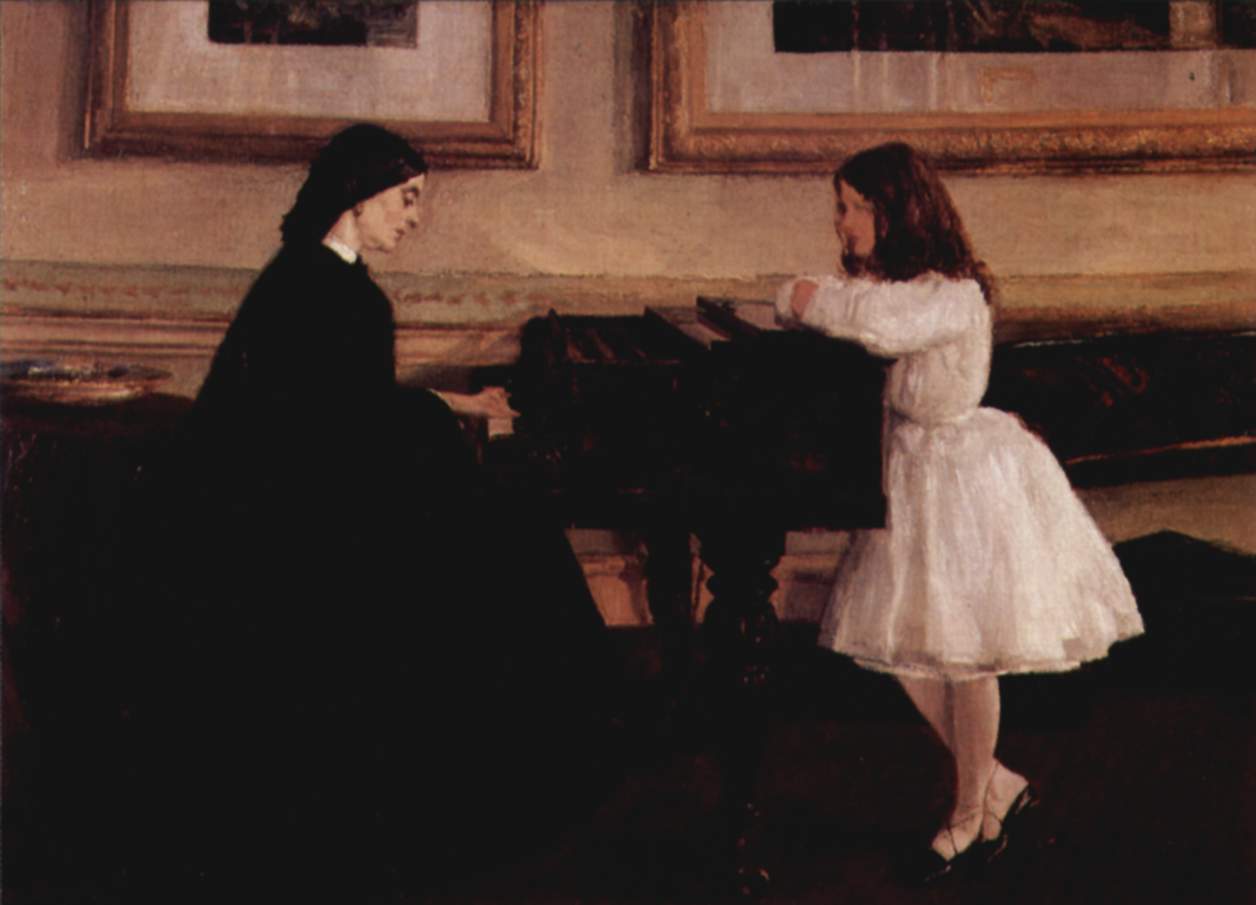The image portrays an interior setting of an older-style building, likely from the late 1800s, depicted in a detailed painting. The background features light beige or tan walls with large, ornate framed pictures hanging, though the specifics of these pictures are not clear. The floor is tan, with the bottom of the wall appearing brown, resembling wood, and a dark rug or carpet underneath a black piano.

At the center of the painting, a woman dressed in a voluminous black robe with a white piece around her neck is seated at the piano. Her light-skinned hands are gracefully stretched out over the white piano keys, and her dark hair is pulled back over her neck. It suggests a somber or formal atmosphere, possibly indicating she is a nun or in mourning.

Standing to the right of the piano is a young girl clad in a white dress that reaches her knees, accentuated by white stockings and black slippers. Her dark brown, slightly reddish-tinted hair cascades over her shoulders. She is intently observing the woman playing the piano, her gaze fixed on the musician. The detailed depiction of their clothing and surroundings emphasizes the artistic and historical nature of the scene.